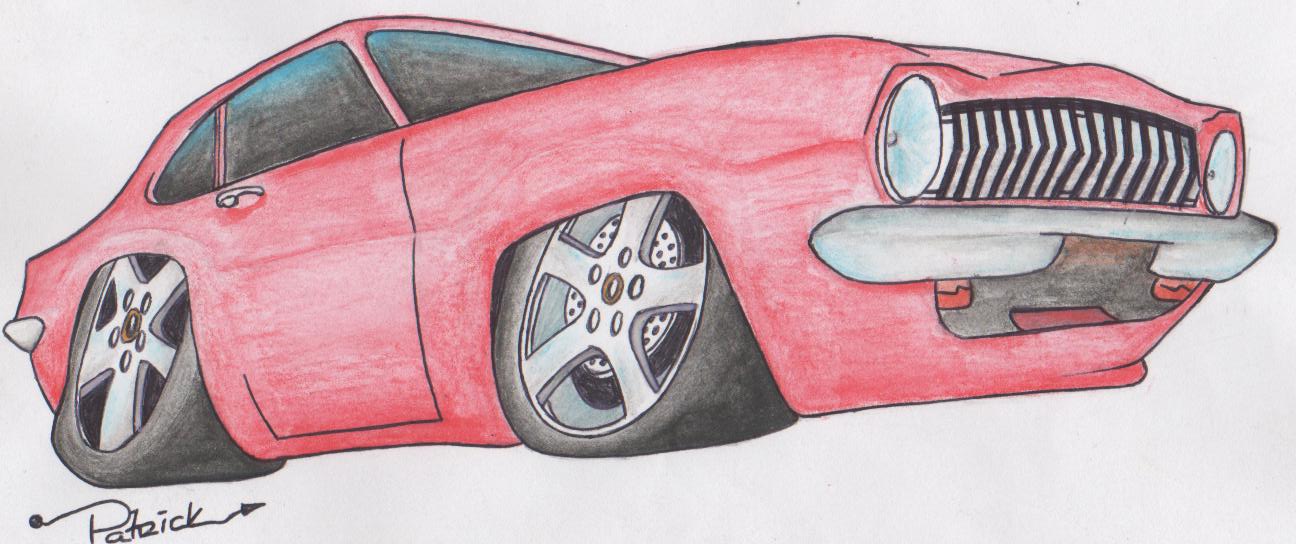This image is a detailed, colored pencil drawing of a vintage-style red sports car, possibly resembling a classic Mustang. The car is depicted from a slightly angled side view, facing right, on a plain white paper background with no additional scenery or detail. The red body of the car is smoothly shaded without any decorative paint stripes. It features black tires with simple steel rims, wide tires that almost appear to melt into the ground, and a chrome bumper and grille. The headlights are classic round styles, similar to those found on old motorcycles, and the windows are tinted black. The car has chrome door handles and a visible silver exhaust pipe. In the bottom left corner of the drawing, the artist's signature "Patrick" is inscribed, with unique detailing where the "P" has a circle and the "K" features an arrow-like extension.